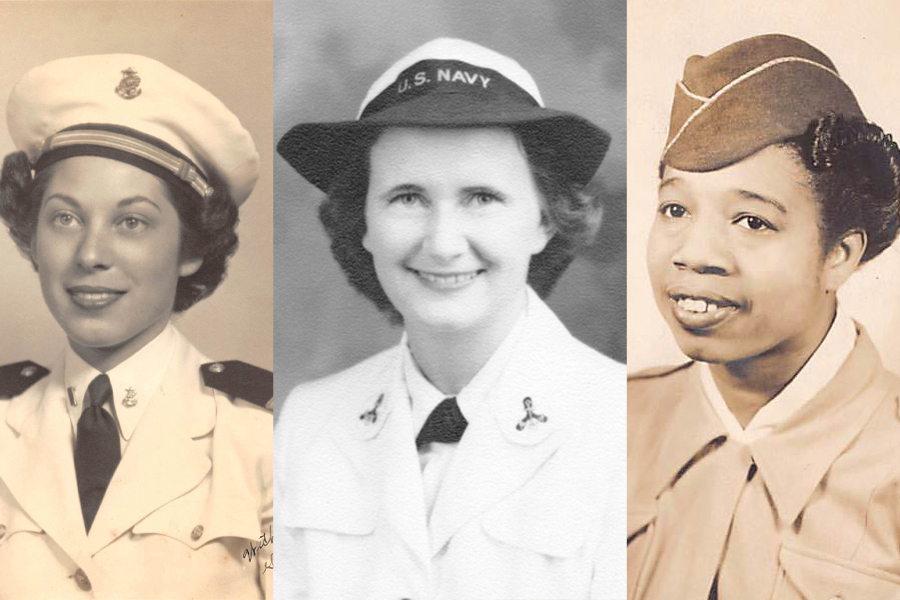This image is a side-by-side montage of three sepia-toned and black-and-white photographs featuring women in different branches of the U.S. military from an earlier era, likely mid-20th century. Each photograph showcases a young woman, estimated to be between 20 and 28 years old, all smiling confidently.

The woman on the left, dressed in a sepia-toned Marine Corps uniform, sports a dress white hat with a prominent Marine Corps emblem, along with a black tie and buttoned front pockets. She has short, curly hair and her lapels display the Eagle, Globe, and Anchor insignia, likely indicating a rank of First Lieutenant or Captain.

The middle image in traditional black and white features a Caucasian woman in a U.S. Navy uniform with a distinctive, almost floppy hat marked "U.S. Navy." She has a short ascot-type tie and decorations on her collar. Her genuine smile further accentuates her neatly arranged dress whites.

The woman on the right, an African-American, wears an Army or Navy banana-style cap with white piping. Her outfit comprises a tan or white shirt with buttoned flap pockets but no tie, and her short black hair is neatly pinned back. Despite the lack of clear branch identification, her attire signifies military service.

These vintage photos collectively portray the diverse roles women have played in U.S. military history.